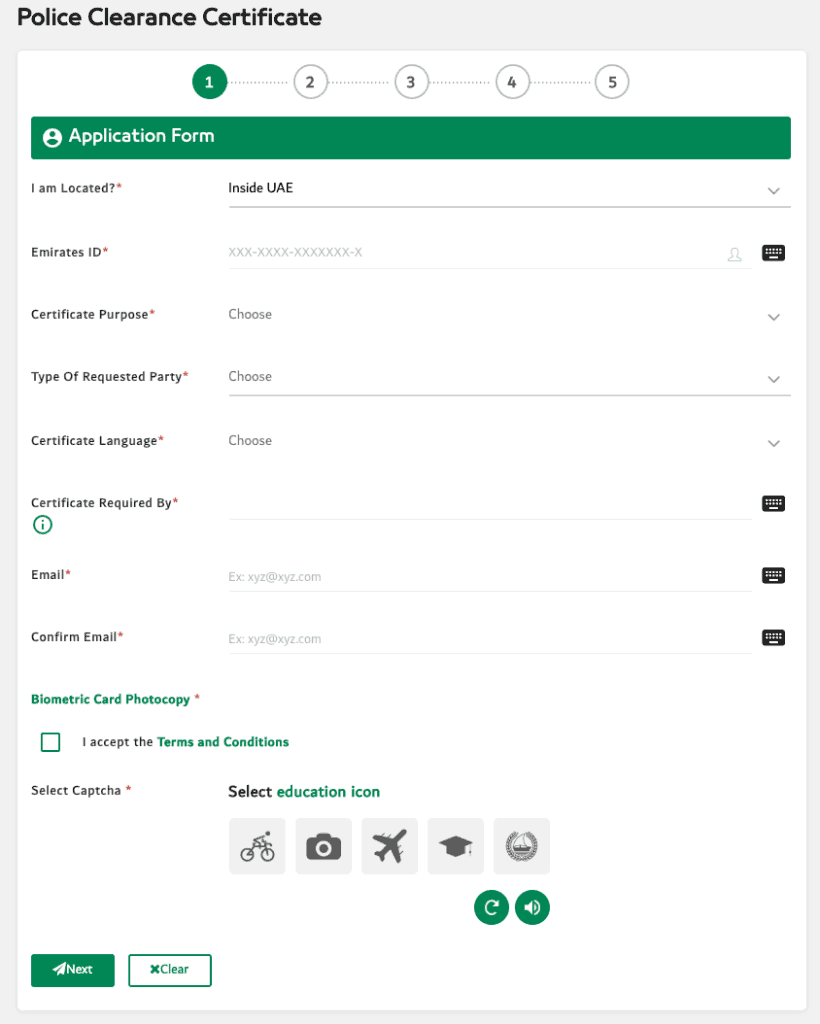The image displays a webpage for obtaining a Police Clearance Certificate. At the top-left corner, there is a prominent title in bold, "Police Clearance Certificate". The page has a light gray border that frames the content. Below the title, there is a series of five numbered circles. The first circle is green with a white number "1" inside it, while the remaining circles are white with black numbers.

Directly beneath the circles, a green banner is present, featuring a profile icon on the left, followed by the words "Application Form" towards the right. Under this section, a question is posed with "I am located" followed by a red star, suggesting a mandatory field. To the right of this, the options "Inside UAE" appear adjacent to a drop-down arrow, separated by a line. Further left, there is another section denoted with "Emirates ID" accompanied by a red star, alongside a small keyboard icon.

The subsequent part of the form includes fields for "Certificate Purpose", "Type of Requested Party", "Certificate Language", "Certificate Required By", followed by "Email" and "Confirm Email", all marked with red stars indicating required fields. Below these fields, there is a section for "Biometric Card Photocopy" with a corresponding upload box.

Near the bottom of the form, there is a checkbox for accepting the terms and conditions. Further below, instructions prompt the user to select a CAPTCHA and an education icon, with five icons displayed for this purpose. Finally, at the bottom of the page, there are two buttons: "Next" for proceeding with the application and "Clear" for resetting the form.